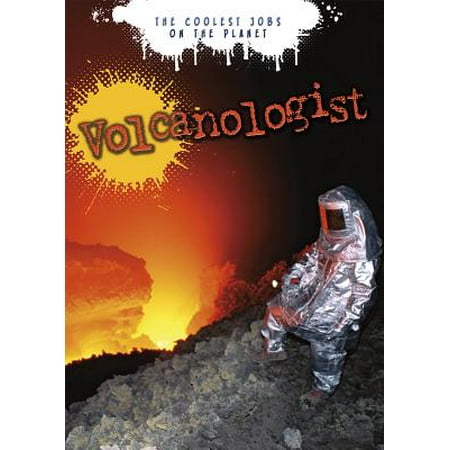The image captures a dramatic scene of a volcanologist standing on the rocky ground near the edge of an active volcano, positioned on the far right side of the image. The volcanologist is fully geared in a reflective silver heat-resistant suit with a face shield, making it impossible to see the person inside. The background showcases an intense display of natural forces, featuring an orange and yellow volcano emitting bright lights, steam, smoke, and fiery sparks. The top portion of the image presents the text "the coolest jobs on the planet" in black letters within a dripping white cloud-like shape. Below this, the word "volcanologist" is prominently displayed in orange text across the image, with a yellow circular splatter emitting sparks near the left side around the letter 'V'. The volcanic landscape also includes splashes of red and black, suggesting the presence of lava and magma. The overall color scheme includes shades of black, red, orange, yellow, gray, and silver, contributing to the image's vivid and dynamic atmosphere.